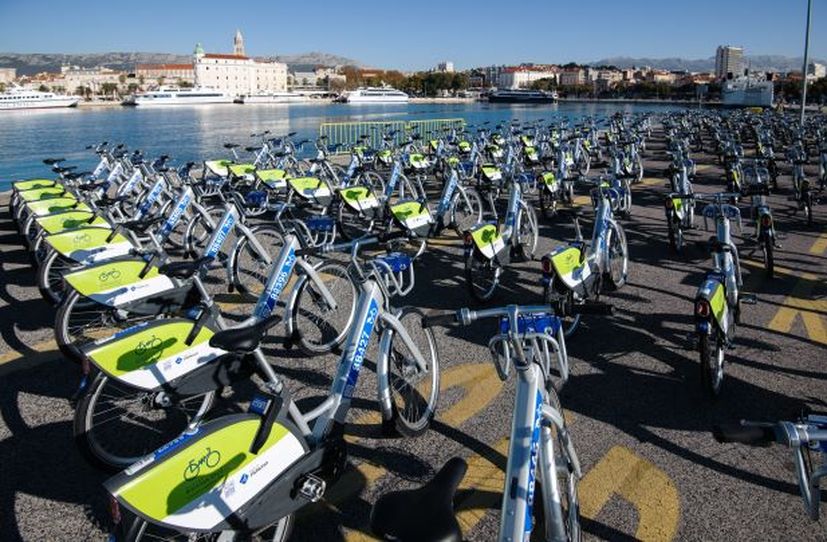This photograph, taken in an outdoor setting during the morning, captures a well-organized parking lot filled with a multitude of blue and grey bicycles, which are likely part of a city bike rental service. Each bike has a black seat and features a green and white promotional label that indicates ownership by the city, possibly for tourists and locals to rent for exploring downtown areas. The concrete ground beneath the bicycles, which is marked with some yellow spray paint, shows shadows cast by the morning sun. On the left side of the image, a river with clear blue water can be seen, populated by large white yachts and ships. Across the river, a line of buildings, which appear to be tall, older structures with many windows, possibly hotels, rise against a backdrop of distant mountains. The entire scene is set under a clear blue sky, indicating a bright and pleasant morning, potentially in a tourist-friendly locale resembling coastal areas in Italy or France.